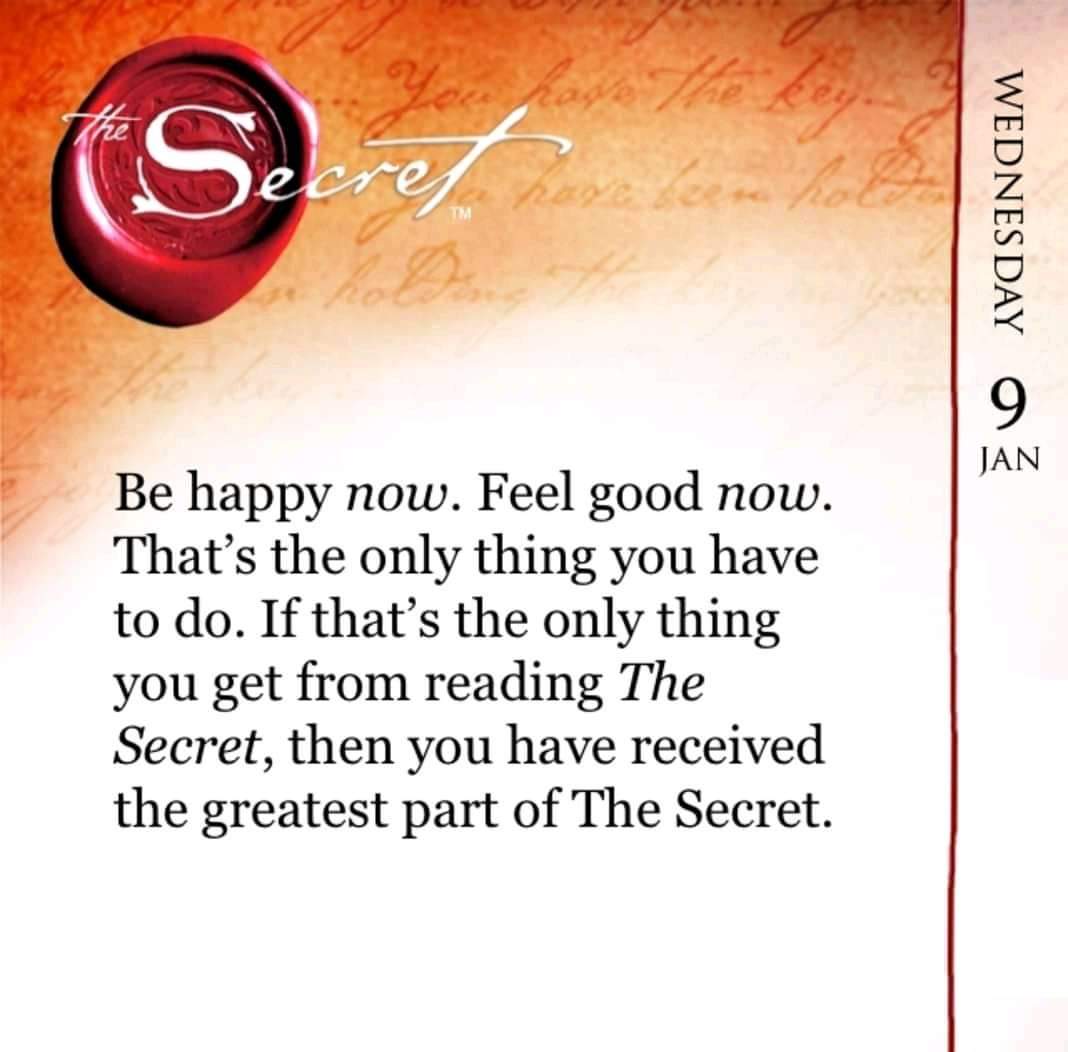This image, featuring an excerpt from the book "The Secret," presents a visually rich and detailed page. In the upper left corner, a red-colored wax seal embeds the logo of "The Secret," with the title written in white font on an orange-hued background. The background resembles aged parchment, adorned with faint, handwritten script. Vertically aligned on the upper right, the date "Wednesday, 9th January" is marked, separated by a red border. At the center, the focal point is an inspirational quote printed in black letters on a white background, which reads: "Be happy now. Feel good now. That is the only thing you have to do. If that's the only thing you get from reading 'The Secret,' then you have received the greatest part of 'The Secret.'" This page encapsulates a primary message from the book, set within a visually thoughtful design.